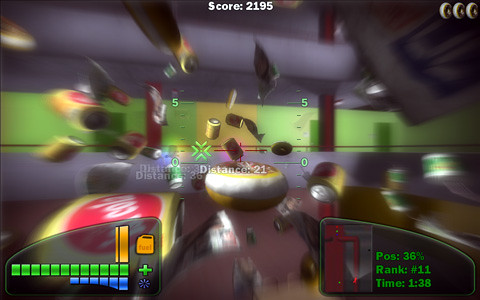This is a screen grab from an in-action video game, possibly on a computer or console. The image is somewhat blurry, indicating motion, making it difficult to discern all details. In the background, there is a green wall with a yellow accent in the center. Various objects, maybe cans of soda or cat food, are flying through the middle of the air in different colors like yellow, red, and green. In the top left corner, there is a character with a green square base, yellow limbs, and a triangular head. The center of the screen features a donut-shaped object coming towards the viewer and a green crosshair with "Distance 21" next to it. The top of the image displays the score "2195" in white lettering, with three donut-shaped icons in the upper right corner that might represent lives. The bottom right shows in green text: "Position 36%, Rank 11, Time 138." On the left side, there are small screens indicating character health: a yellow bar next to a yellow fuel can labeled "fuel," a green bar beside a green plus sign, and a blue segmented bar next to a blue asterisk.